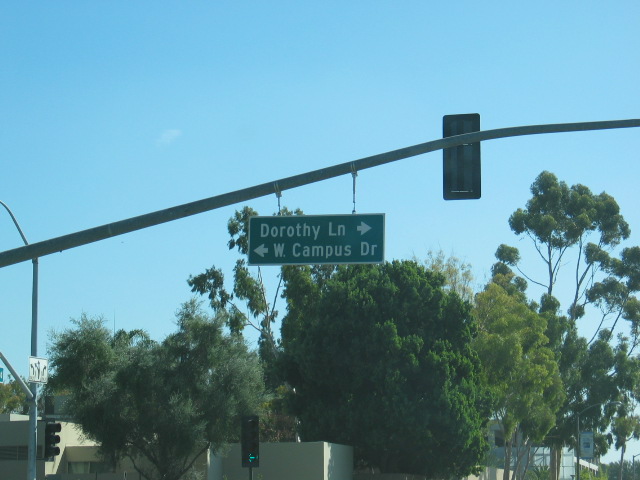This is a square color photograph of a street scene featuring a prominent street sign and multiple traffic lights set against a bright, clear blue sky, typical of a warm climate like Los Angeles. The primary street sign hangs from a long, gray steel pole in the middle of the frame, displaying "Dorothy Lane" with a rightward white arrow, and below it, "West Campus Drive (W Campus Dr)" with a leftward white arrow. The photo's upper portion showcases an expanse of blue sky with only one visible cloud. To the right of the main street sign, we see the backside of a traffic light or sign. Amidst the vibrant foliage in the scene, there is a mix of tree types: a tall, slim tree on the right, a bushy dark green tree in the center, and a tree resembling an olive tree on the left. Additional details include another traffic sign and light in the lower left-hand corner, providing turn directions, and modern white and tan stone buildings visible in the lower right-hand corner.